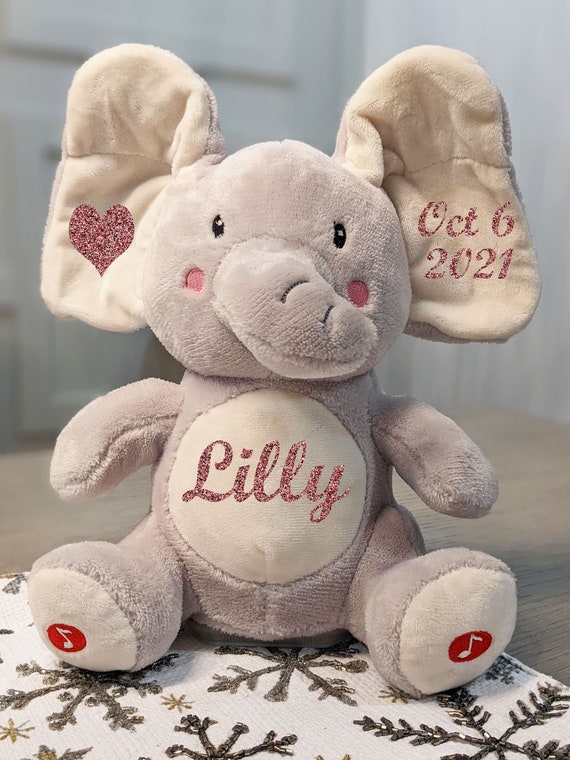This detailed photograph captures a charming light grey stuffed elephant sitting on a tabletop, laid atop a blanket embroidered with snowflakes. The elephant, adorned with numerous personalized details, features black shiny eyes and two pink circles on its cheeks that add to its adorable expression. Its belly displays a white circle with the name 'Lily' written in glittery pink letters. The elephant's distinctive ears further enhance its uniqueness: the left ear showcases a glittery pink heart, while the right ear is marked with the date "October 6, 2021" in the same glittery pink writing. The elephant’s feet are white, each adorned with a red circle containing a white music note icon, making this stuffed toy not only a cuddly companion but a truly special keepsake.